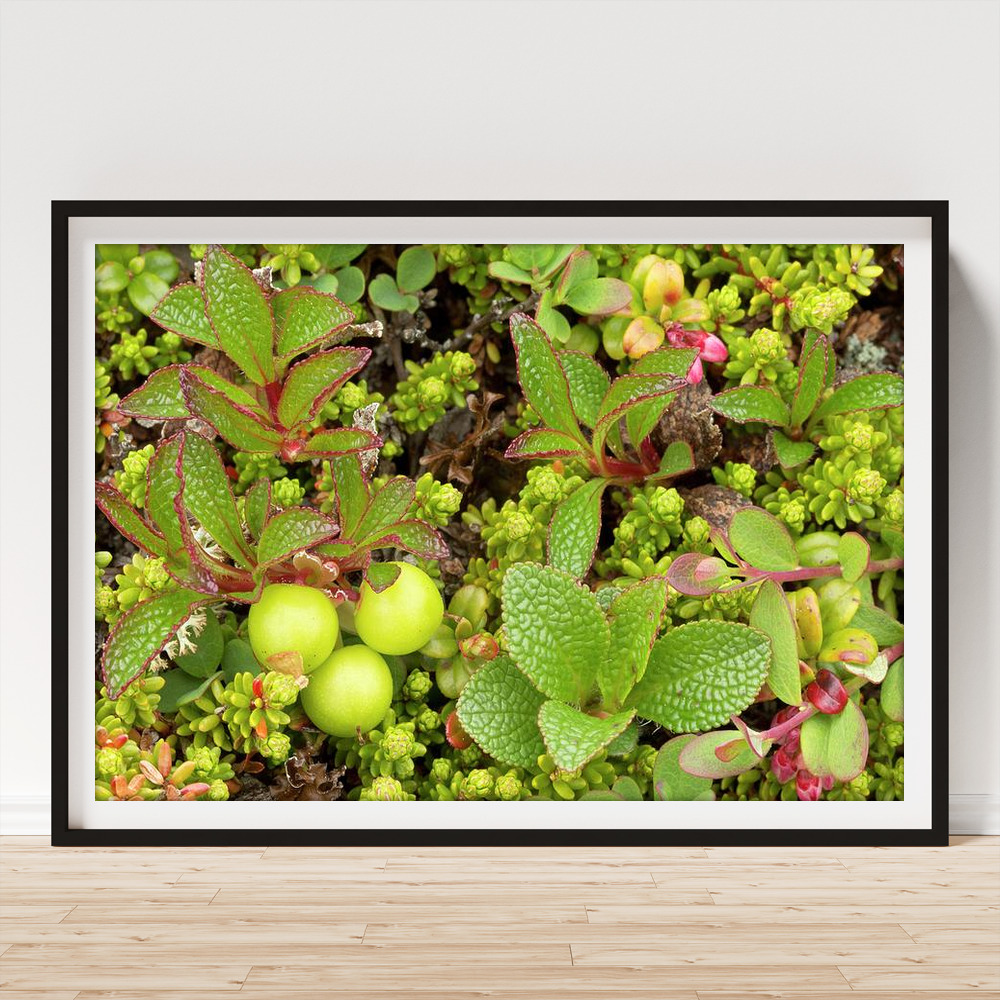The image portrays a framed photograph of diverse plant life, propped up against a light blue wall on light brown wooden flooring. The frame features a black outer border and a white inner border, framing the vibrant close-up of various plants. Prominently, on the left side, a leafy green plant with violet-trimmed edges showcases three green berries or fruit. Similar foliage appears towards the top right, though without any fruit. The photograph is rich with textured leaves, some with pink or purple ends, and displays a colorful array of green, purple, and yellow hues, capturing an intricate and lively botanical scene.